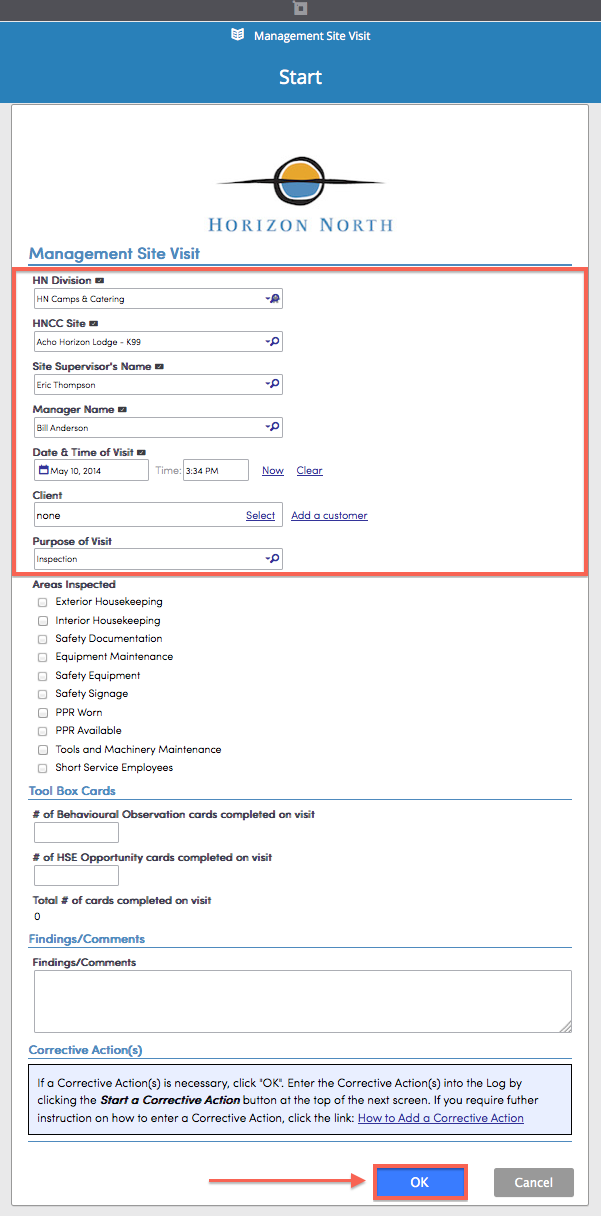The image depicts a detailed form for documenting a management site visit at Horizon North, part of their Camps and Catering division. The form's layout is structured as follows:

1. **Header**:
   - "Management Site Visit, Start" is prominently highlighted in white against a blue background.
  
2. **Company Information**:
   - The Horizon North logo is displayed with the accompanying text "Management Site Visit".

3. **Site and Supervisor Details**:
   - **HN Division**: "HN Camps and Catering" (with a drop-down menu).
   - **HNCC Site**: "ACHO Horizon Lodge-K99" (with a drop-down menu).
   - **Site Supervisor**: "Eric Thompson" (with a drop-down menu).
   - **Manager Name**: "Bill Anderson" (with a drop-down menu).
   
4. **Visit Information**:
   - **Date and Time of Visit**: May 10, 2014, at 3:34 p.m. Options for "Now" and "Clear" are available.
   - **Client**: "None" (with an option to add a customer via a highlighted blue hyperlink, "Add a Customer").
   - **Purpose of Visit**: "Inspection" (with a drop-down menu).

5. **Areas Inspected**:
   - Includes checkboxes for various inspection areas such as exterior housekeeping, interior housekeeping, safety documentation, equipment maintenance, safety equipment, safety signage, PPE worn, PPE available, tools and machinery maintenance, and short service employees. None of these boxes are currently checked.

6. **Toolbox Cards**:
   - **Number of Behavior Observation Cards Completed on Visit**: No cards completed (empty box).
   - **Number of HSE Opportunity Cards Completed on Visit**: No cards completed (empty box).
   - **Total Number of Cards Completed on Visit**: Zero.

7. **Findings/Comments**:
   - A large rectangular box for entering findings or comments, which is currently empty.

8. **Corrective Actions**:
   - Instructions for adding corrective actions, including a prompt to click "OK" if necessary. Further instructions are provided via a link titled "How to Add a Corrective Action". At the bottom of this section, a red arrow points to an "OK" button next to a "Cancel" button.

This detailed and structured form ensures thorough recording and follow-up of management site visits at Horizon North sites.